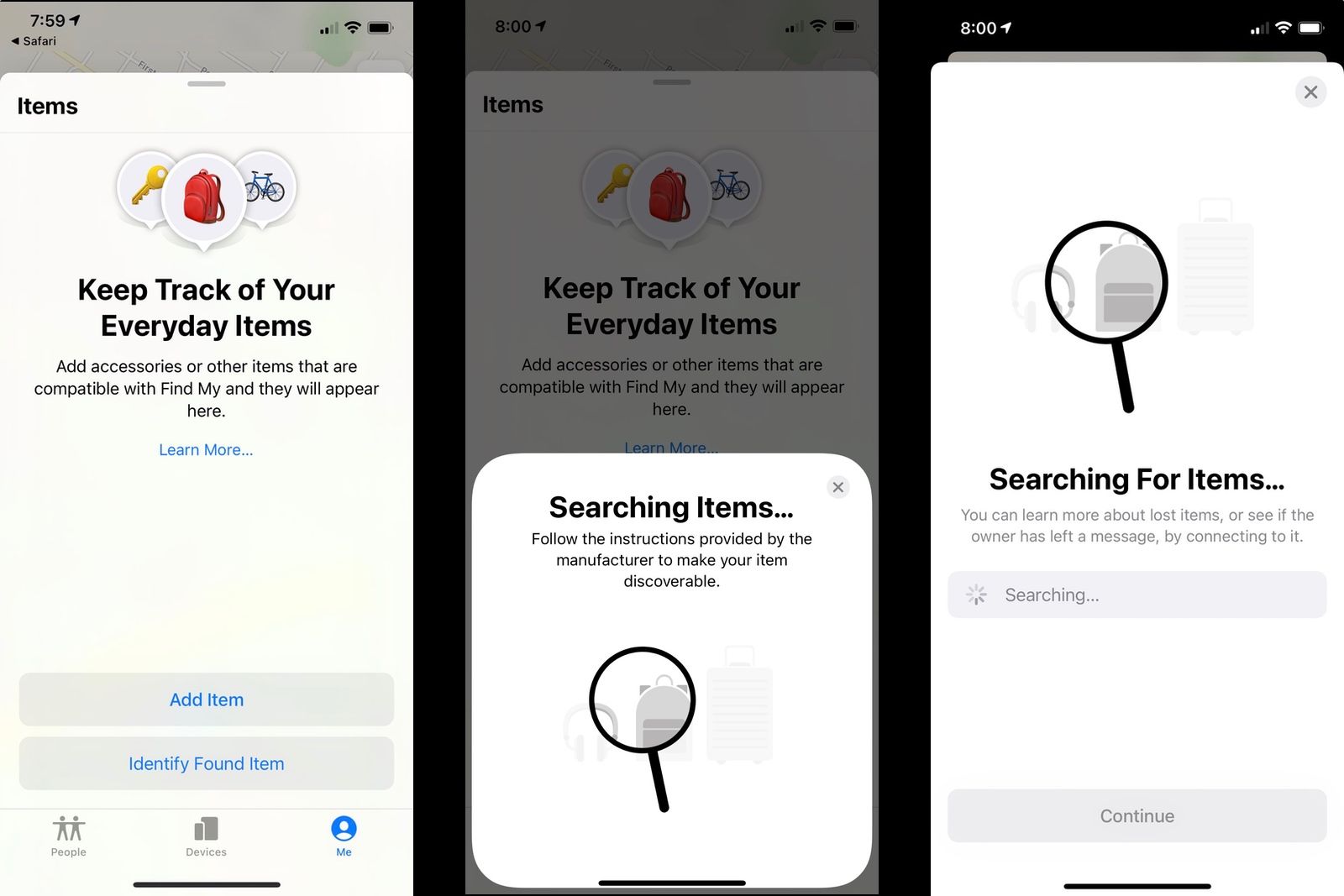This is a detailed screenshot captured on an iPhone, evident from the recognizable Safari Explorer icon. The first screen features a tracking app, prominently titled "Keep Track of Your Everyday Items." This screen likely serves as the app's main dashboard or homepage. Transitioning to the second screen, the interface displays a "Searching Items" dialog box, accentuated by a magnifying glass icon, suggesting that the user has initiated a search query. The third screen showcases a more expanded "Search for Items" tab, indicating active progress in locating specific items, although the exact purpose or functionality of the app remains unclear without prior experience using it.